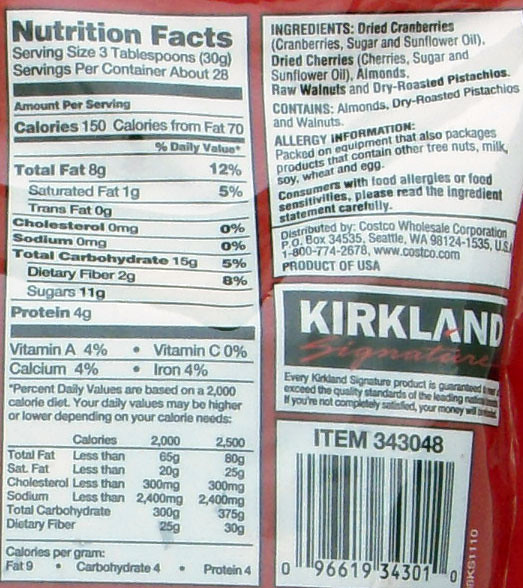The image displays the back of a shiny, reflective red bag of a Kirkland Signature product, predominantly displaying the nutrition facts and ingredients. The nutrition facts section, outlined in black, occupies a large vertical strip on the left side of the image, featuring details such as serving size (3 tablespoons), servings per container (28), and calories per serving (150). It also lists nutritional content, including 12% total fat, 5% total carbohydrates, 8% daily fiber, and 4 grams of protein, along with vitamins A and C, calcium, and iron. Next to it, on the right side, is a smaller white box containing the ingredients: dried cranberries, dried cherries, almonds, raw walnuts, and dried roasted pistachios. Allergy information is noted due to the nut content. Below the ingredients, the Kirkland Signature logo is prominently displayed in black and white, with the signature in red. Beneath the logo is the barcode and item number, aiding in product identification. The packaging overall conveys a detailed breakdown of the product's nutritional value and components, consistent with a high-quality trail mix distributed by Costco Wholesale Corporation.